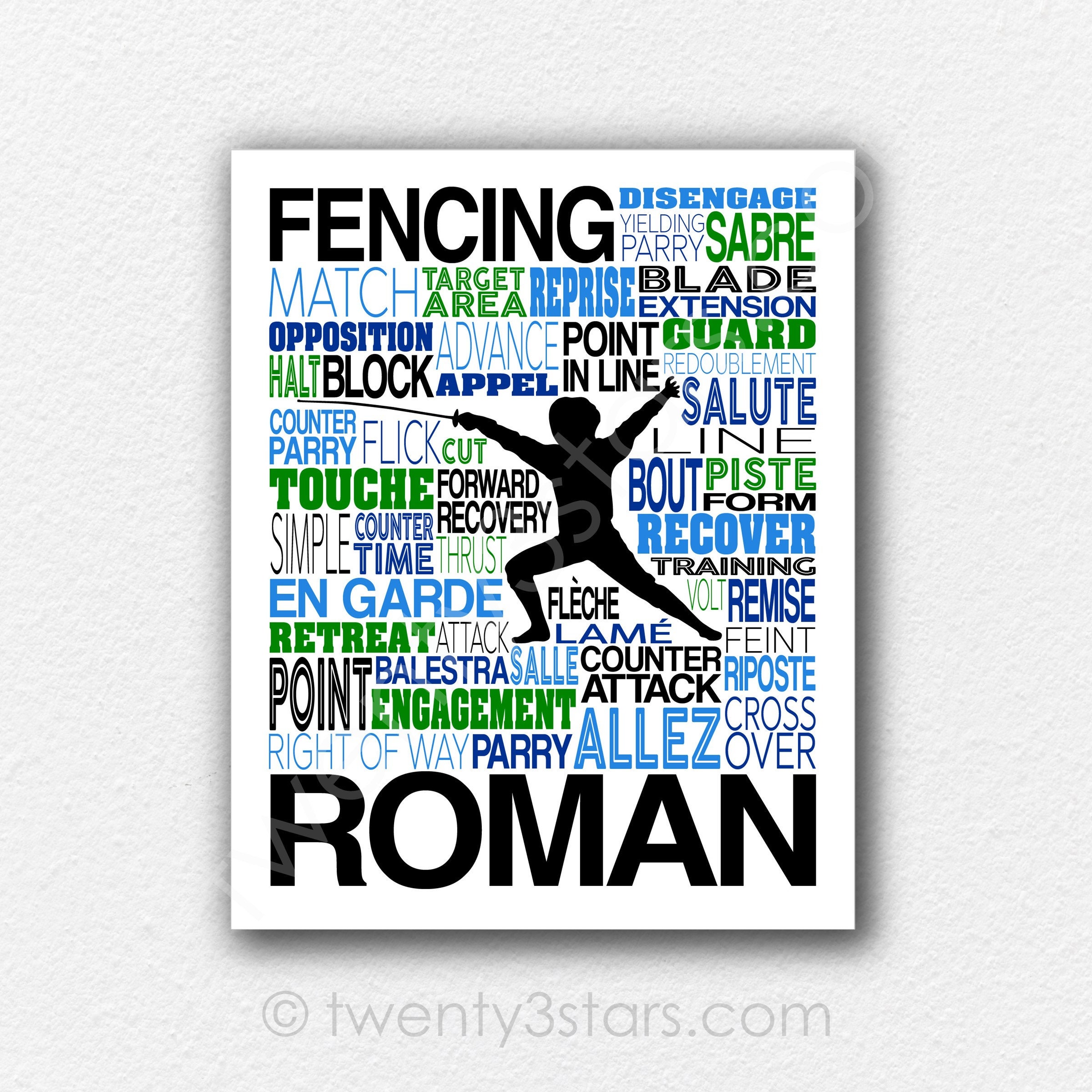The image appears to be a square, poster-sized advertisement on a grey background, featuring a prominent white square. In the center, there is a silhouette of a fencer in an action pose, holding a thin fencing sword. The top left prominently displays the word "Fencing" in large letters, while the bottom showcases "ROMAN" in uppercase black letters. Surrounding the fencer are various fencing-related terms in different fonts and colors, such as blue, black, and green. These words include "disengage," "parry," "yielding," "saber," "blade," "extension," "recover," "training," "salute," "counter-time," and "touche." At the very bottom, in a lighter color, it reads "see in a circle 23stars.com." The entire composition emphasizes the dynamic art and vocabulary associated with fencing.